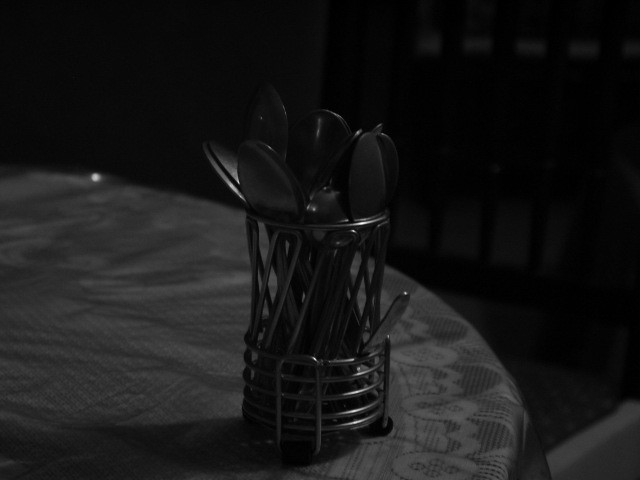The image is a black and white close-up of a metal wire container containing silverware. The spoons, which are placed with their heads facing upwards, form a prominent cluster, mostly in silhouette due to the very dark lighting. Alongside the spoons, a knife and another utensil handle protrude from the container. The container is positioned on the edge of a circular table adorned with a patterned tablecloth in varying shades of gray and black. The background fades into the dark setting, leaving the silverware and parts of the table as the main visible elements in the composition.